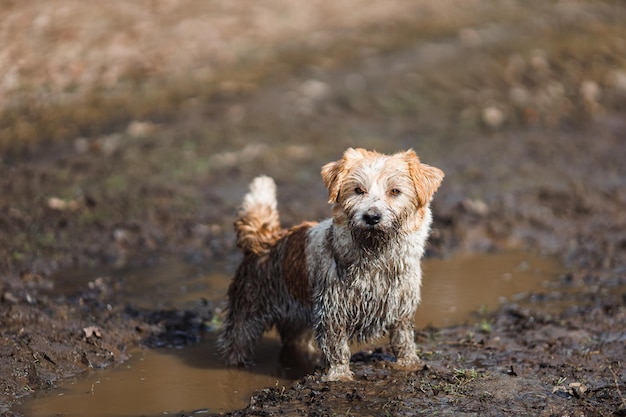This photograph captures a small dog with shaggy, tricolor fur featuring beige, brown, and white patches. The dog is outside, standing in a narrow oval puddle of brown, muddy water. Its back paws are submerged in the puddle while its front paws rest on drier mud. The dirt ground beneath the dog is blurred in the background but clear in the foreground, emphasizing the wet, muddy texture. The dog's grayish fur is matted with mud spots, blending seamlessly with the muddy surroundings. The dog has brown eyes and a big black nose, with distinctive features resembling a Shih Tzu or terrier mix, including what appear to be furry eyebrows. With its ears down and tail up, the dog looks directly at the camera, conveying a mix of curiosity and slight dismay, as if acknowledging its muddy escapade. The background remains indistinct, keeping the focus entirely on the mud-covered dog and its gritty environment.